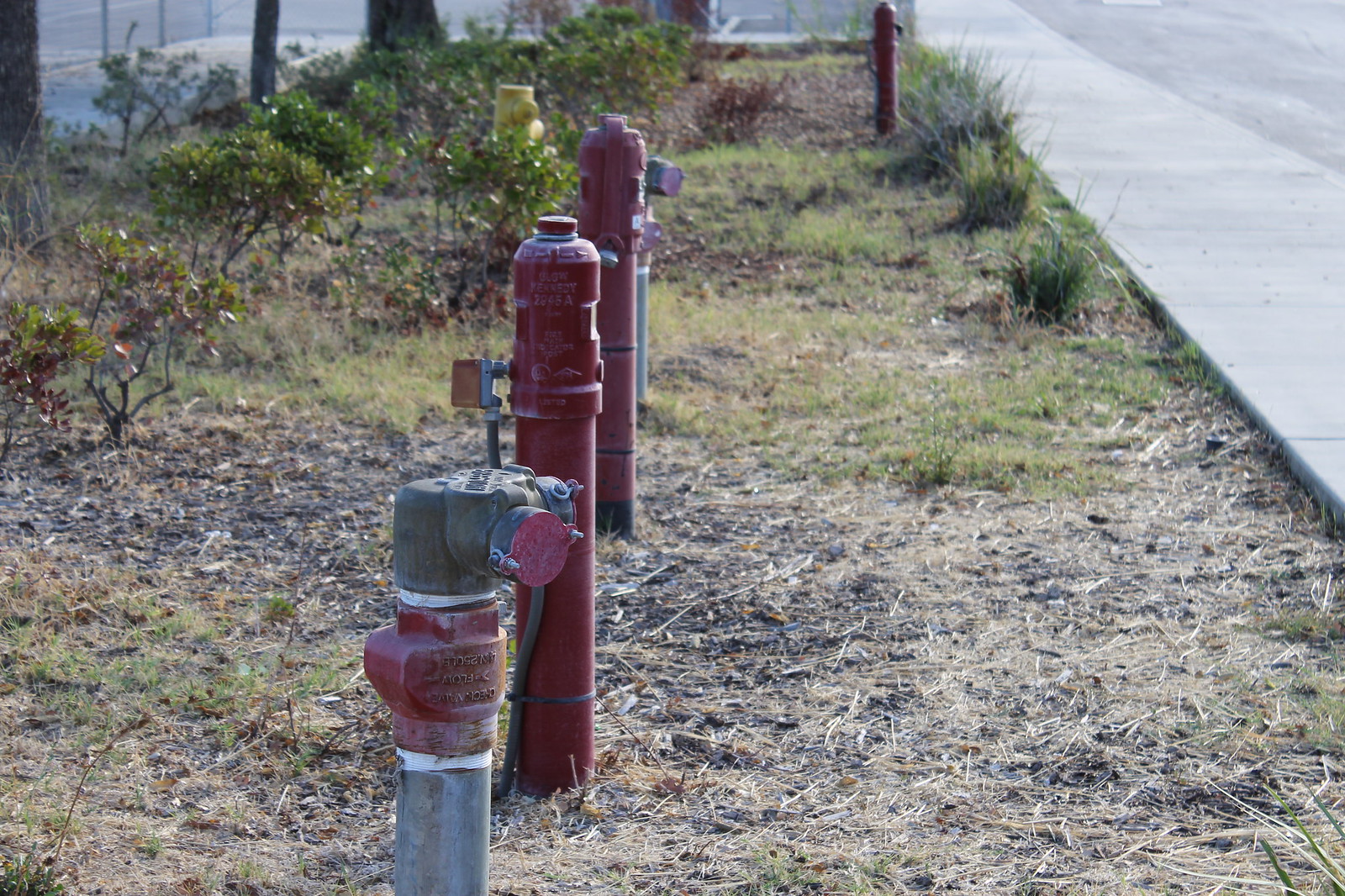The image depicts an outdoor scene situated in a large green space between two streets. In the center of this area, three tall, slender metal pipes stand prominently, each with distinct features and colors. Two of these pipes are identical and painted a deep red, while the third pipe, positioned towards the front of the image, is primarily gray with a red center and has two extensions that look adjustable, potentially for attaching hoses. The pipes appear to be somewhat weathered, with chipped paint exposing the underlying metal.

The ground around these pipes is a mix of beige dirt and patches of unkempt grass interspersed with twigs. To the right, a gray sidewalk runs parallel to the green space, with a small segment of the adjacent street visible. Behind the pipes, a yellow fire hydrant is discernible, with some scrubby plants and green shrubbery filling in the background. The vegetation surrounding the pipes includes almost dead grass and green patches, which add to the overall rough and untended appearance of the area. The scene suggests the pipes might be part of a utility system for water or gas, given their accessibility and structure.